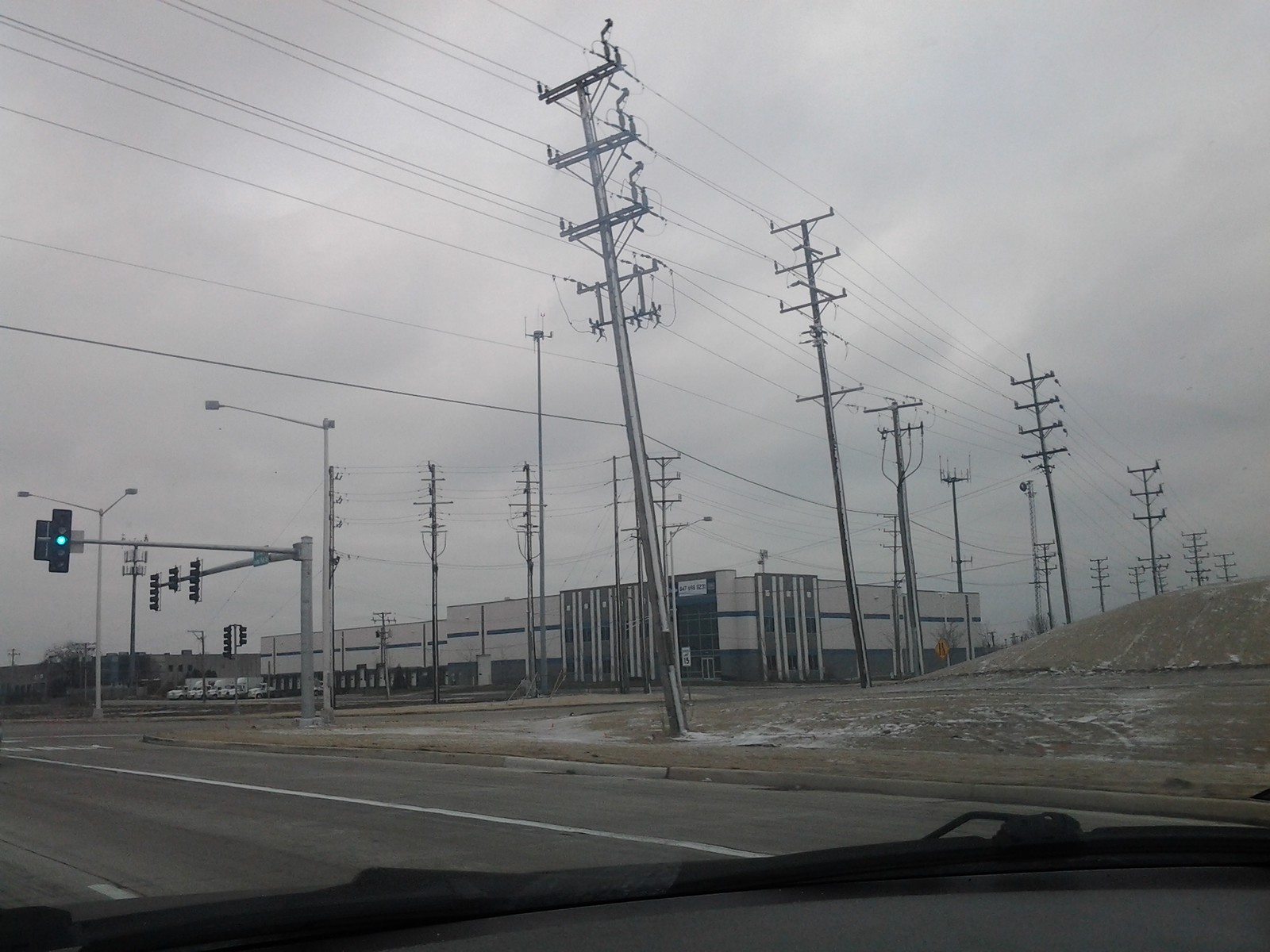This black-and-white photograph captures an expansive, desolate industrial landscape on a gray, cloudy day that appears ominous and stormy. In the foreground, a road approaches an intersection with a traffic light showing green. The road spans from the bottom right to the bottom left of the image, suggesting the photo was likely taken from inside a vehicle, as the bottom of the windshield and a windshield wiper are visible. Dominating the scene are large metal power lines, which crisscross the sky with three or four tiers of wires, suggesting proximity to an electrical facility or power distribution center. The backdrop features a sizable white industrial building with some blue decorative accents and an adjacent flat area scattered with semi-trucks, highlighting the building's enormous scale. Adding to the bleakness, the landscape includes a hilly, grassy area to the right, nearly devoid of trees or vegetation, and possibly featuring pooled water or snow. The overall atmosphere is one of industrial isolation, further accentuated by the absence of any significant greenery or urban activity.